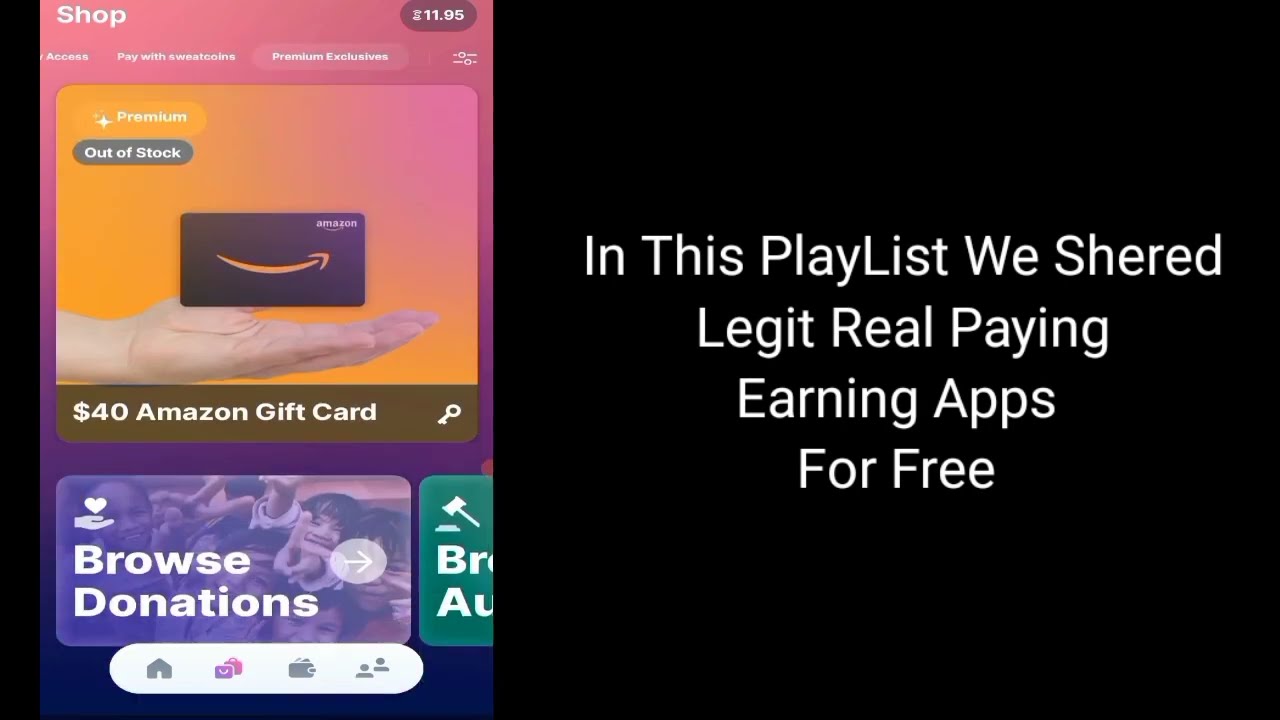The image is an advertisement for an Amazon gift card. On the right side, against a black background, white text reads, "in this playlist we shared legit real-paying earning apps for free," with "shared" misspelled as "S-H-E-R-E-D." In the upper left corner, there's a screenshot with a pink background. At the top of this section, "shop" is written in white letters, with "$11.95" in the upper right corner. Below this, on an orange background, there’s the word "premium" followed by "out of stock" in gray. Underneath, a $40 Amazon gift card is depicted being held by a hand. Below this, a section with a purple background reads "browse donations" and features people in the background, one of whom has a finger pointed upwards. Finally, there's a white-background section with a house icon and other unidentified icons, partially obscured by a green background section showing a hammer and partially visible letters "BR" and "A" and "U."